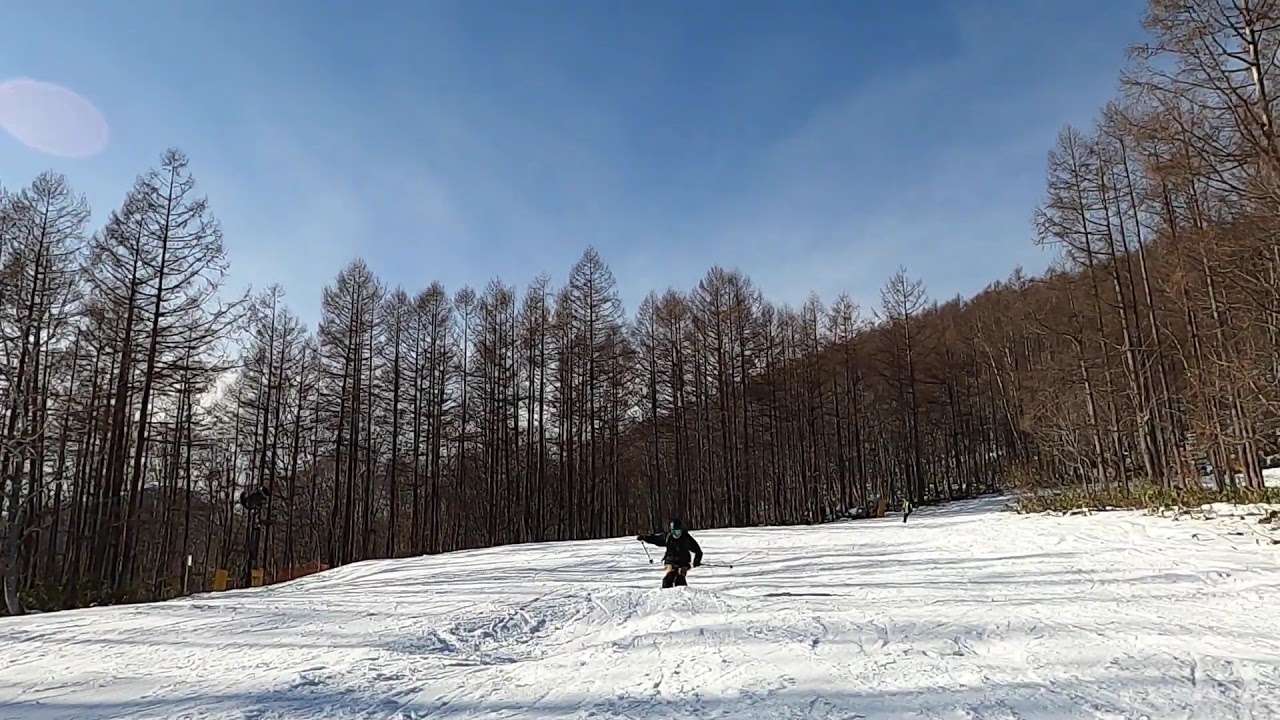A skier clad in a sleek black suit, helmet, and reflective goggles is positioned at the center of a snowy slope, captured mid-descent. The skier grips ski poles in both hands, with the left arm slightly raised and the pole bent back toward the ground, while the right arm is more aligned with the direction of their descent. The snow beneath is crisscrossed with tracks from previous skiers, attesting to a well-traveled route at this ski resort. Tall, leafless trees flank both sides of the slope, framing the action. In the distance, another skier in a light green suit is visible against the backdrop. Further up the slope, a mountain ridge slopes down from right to left, merging with a bright blue sky adorned with hazy clouds. A peculiar white circle is discernible in the upper left corner of the sky, adding a mysterious element to the wintry scene.